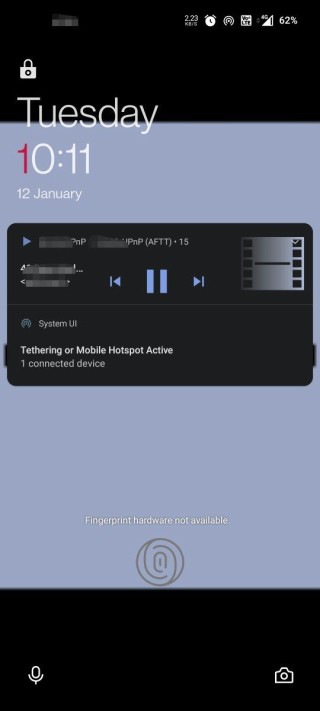A detailed caption for the described image:

"This is a screenshot of a smartphone lock screen. The battery icon at the top right indicates a charge level of 62%. An alarm icon is also visible. At the top center of the screen, the date and time are displayed as 'Tuesday, 10:11, 12th of January,' with the number '10' in red text. Below the time, there is a black notification box with partly obscured text, clearly showing control icons for 'back,' 'pause,' and 'forward.' Additionally, the words 'system' and 'tethering or mobile hotspot active' are discernible, alongside a note stating that one device is connected. The notification overlay background is a blue-teal gradient. Further down, the message 'fingerprint hardware not available' appears, accompanied by a fingerprint icon. At the bottom of the lock screen, there are two action buttons—one for the microphone and one presumably for quick access to the camera. The rest of the screen remains predominantly black."